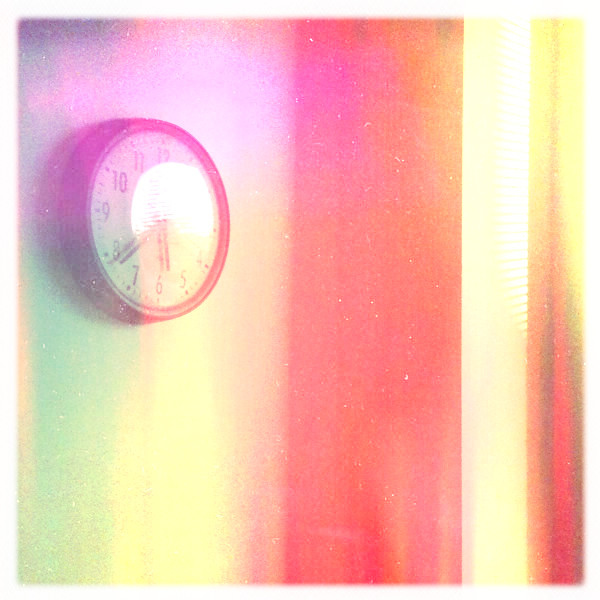A vibrant photograph is overlaid with a rainbow filter, creating a colorful gradient across the entire image. On the left side, a large, round plastic wall clock prominently stands out. The clock features a white face encircled by a bold black ring. Its hour and minute hands are designed with double lines along their outer edges, giving them a striking appearance. The time displayed on the clock is 5:39. The clock has clear, analog numbers marking the hours.

A series of vertical color bands dominate the background, adding to the photo's unique aesthetic. On the far left, a green strip runs downward, followed by a yellow strip. To the right of the yellow strip is a red strip, and adjacent to it, a brighter yellow band appears, illuminated as if light were passing through it. Finally, the last band displays a gradient with yellow at the top seamlessly blending into red at the bottom. The combined elements create a visually compelling image rich in color and detail.